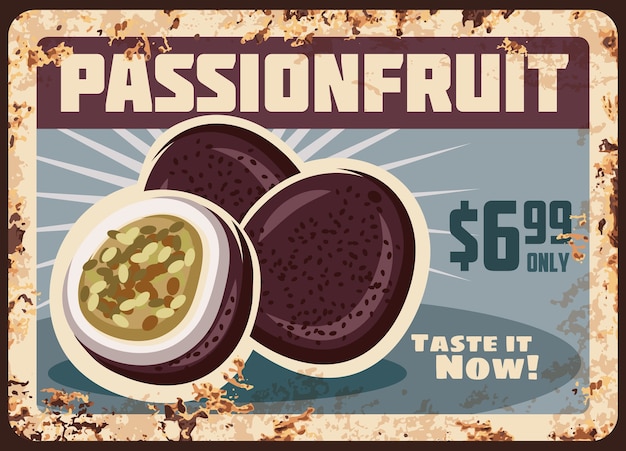This image is a digital advertisement designed to mimic a vintage, rusted metal sign. The rectangular image, approximately four by three inches in size, features a dark border about an eighth of an inch wide, followed by a slightly thicker light tan border with rust-like blotches and rounded edges, evoking an aged aesthetic. 

The header at the top spans horizontally, displaying the words "PASSION FRUIT" in off-white, bold capital letters against a purple background strip. Below this, the main section of the advertisement showcases three cartoon-style passion fruits on a periwinkle blue background. The foremost fruit is cut open, revealing its interior, with white beams emanating from behind the fruits, adding dynamic contrast.

To the right of the illustrated fruits, the text "ONLY $6.99" is prominently displayed in a darker blue, grabbing attention towards the price. At the bottom, inside a darker blue shadowed circle, the enthusiastic call to action "TASTE IT NOW!" is printed in matching off-white, bold font.

Overall, the design emulates a minimalist, simplistic style with added rust effects, capturing the nostalgic feel of an old-fashioned metal plate advertisement.